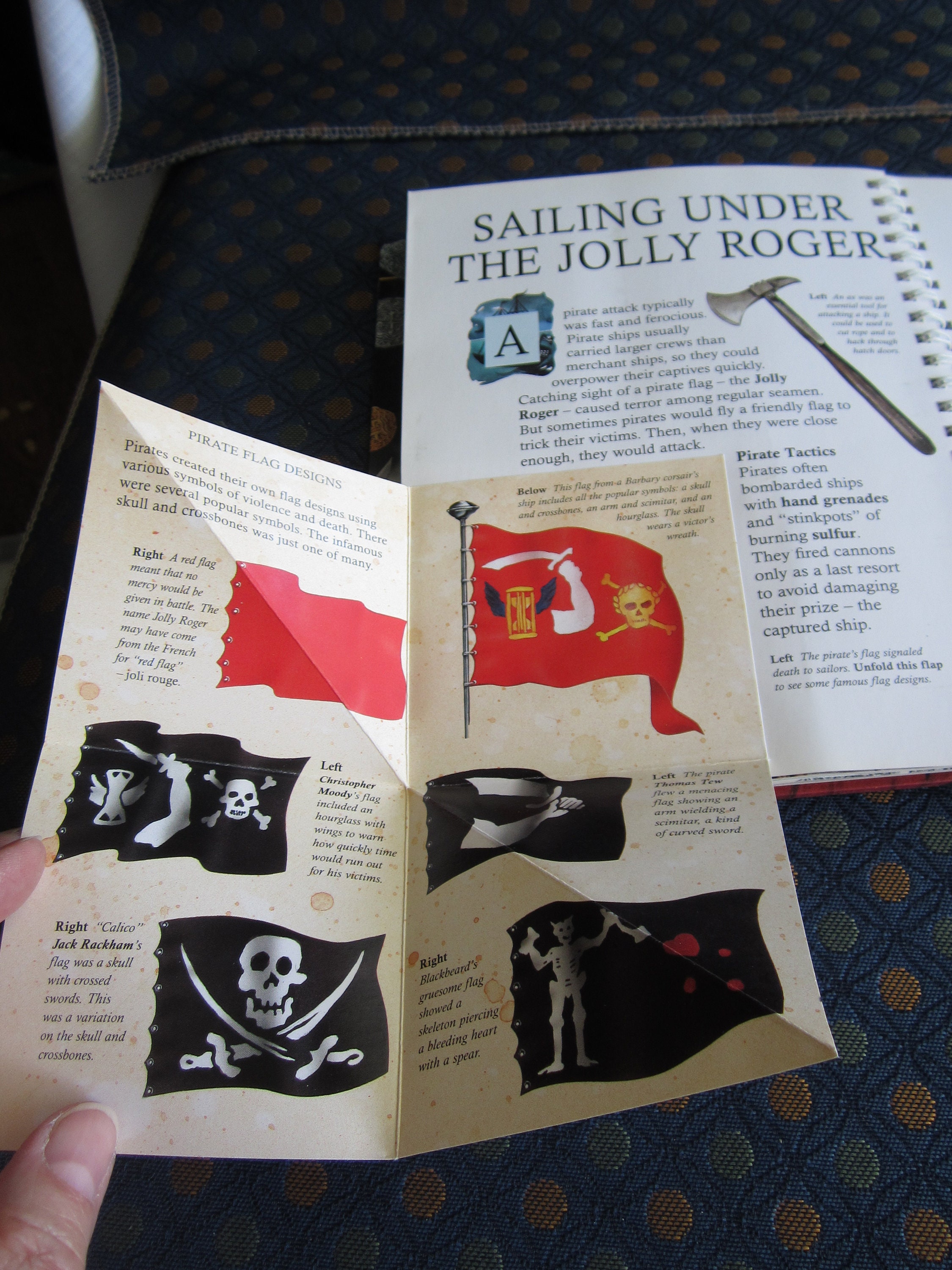In this photograph, a hand holds a paper insert partially unfolded, with an open spiral-bound booklet lying in the background, likely on a bedspread featuring a blue pattern with green and orange spheres interlocked by dark-lined blue rings. The open booklet displays a chapter titled "Sailing Under the Jolly Roger," with text describing pirate tactics and an image of a battle axe. The paper insert, which appears to be made of heavy cardstock resembling old parchment, bears the title "Pirate Flag Designs" and features several pirate flag illustrations. The flags include designs such as a red flag, a skull and crossbones, an arm holding a sword, a skull with crossed swords, and various other menacing symbols. The insert also contains text explaining that pirates created their own flag designs using symbols of violence and death to instill terror. The detailed foldout seems to be affixed to the book on its upper right-hand quadrant, and unfolds dramatically beyond the book's edges, showcasing the intricate and historically inspired flag designs.